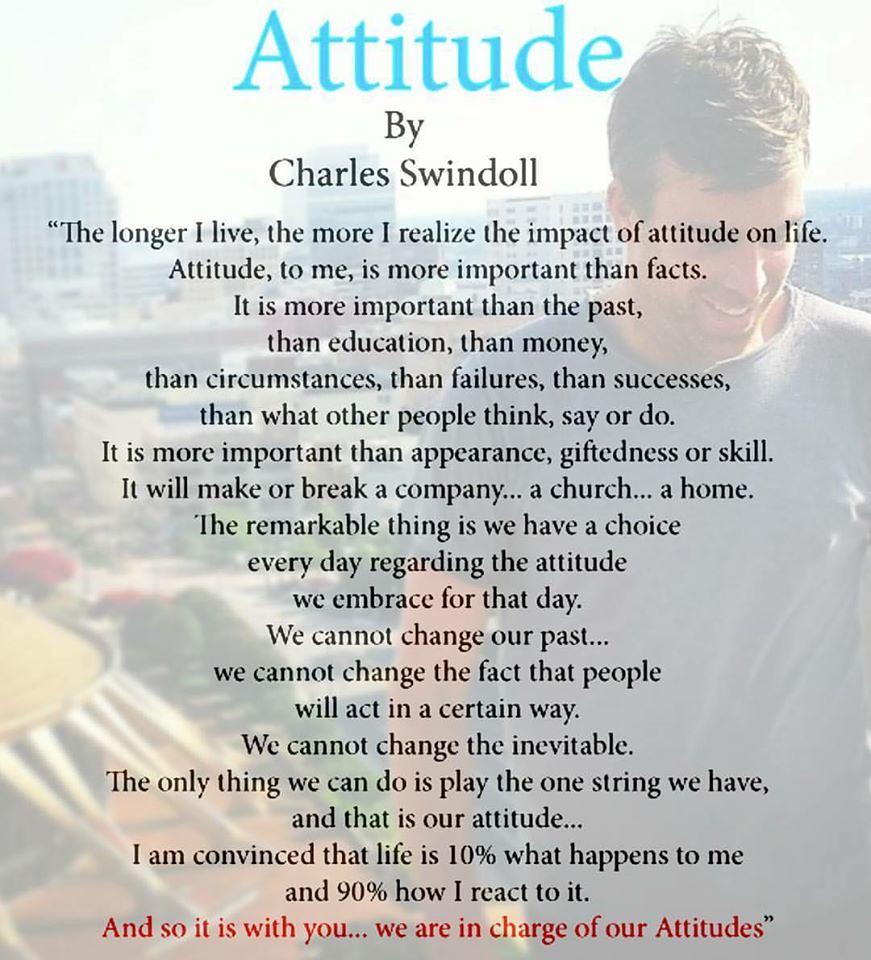The image features a photograph of a man with brown hair, wearing a dark-colored t-shirt, and standing slightly to the right while looking down and smiling against a grayish or white sky backdrop. The overall background also has a gray tint, with a faintly visible city landscape behind him. At the top of the image, the word "Attitude" is prominently displayed in light blue text, followed by "By Charles Swindoll" in black text below. The main body of the text, also in black, reads: "The longer I live, the more I realize the impact of attitude on life. Attitude, to me, is more important than facts. It is more important than the past, than education, than money, than circumstances, than failures, than successes, than what other people think, say, or do. It is more important than appearance, giftedness, or skill. It will make or break a company, a church, a home. The remarkable thing is we have a choice every day regarding the attitude we embrace for that day. We cannot change our past. We cannot change the fact that people will act in a certain way. We cannot change the inevitable. The only thing we can do is play the one string we have, and that is our attitude. I am convinced that life is 10% what happens to me and 90% how I react to it." The text culminates in a highlighted statement in red: "And so it is with you, we are in charge of our attitudes." The image and text collectively convey a motivational message emphasizing the profound importance of attitude in shaping one’s life.